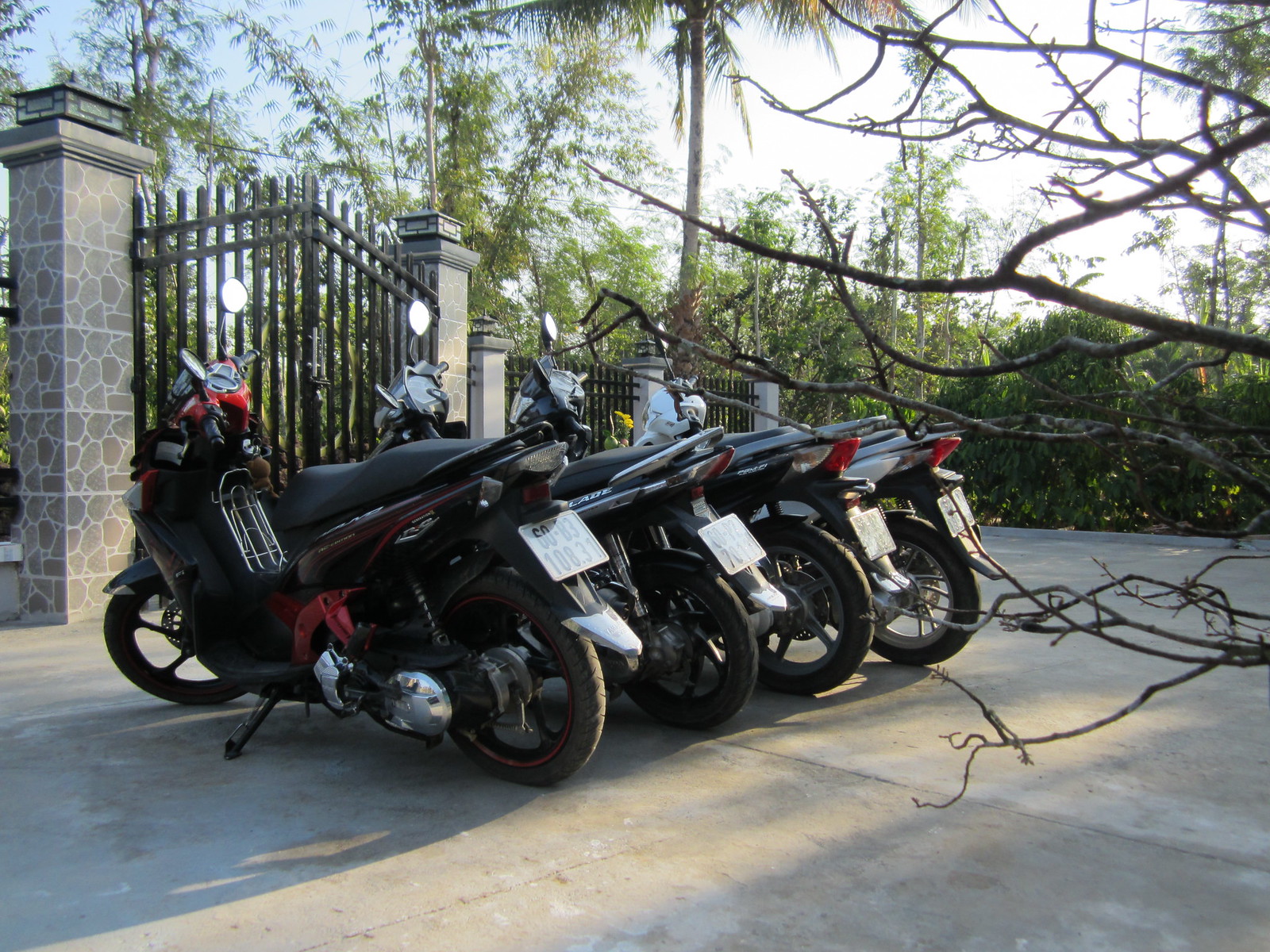The image depicts a row of four sleek, high-speed motorcycles, known as ninja motorcycles, meticulously parked on a grayish concrete surface that resembles a sidewalk in front of a tall, closed gate. The gate is characterized by its imposing stony columns and black wrought iron fence, and there are fallen branches visible on the left side of the ground. The motorcycles, with their distinctly European license plates, are lined up neatly, showcasing subtle differences in color and design. The motorcycle at the forefront stands out with its maroon and red accents, while the following three bikes behind it are predominantly black, with the last one featuring shades of gray. Surrounding the gate are abundant green trees, sparse bushes, and bright branches, set against a light blue sky with sunlight filtering through on the upper right.